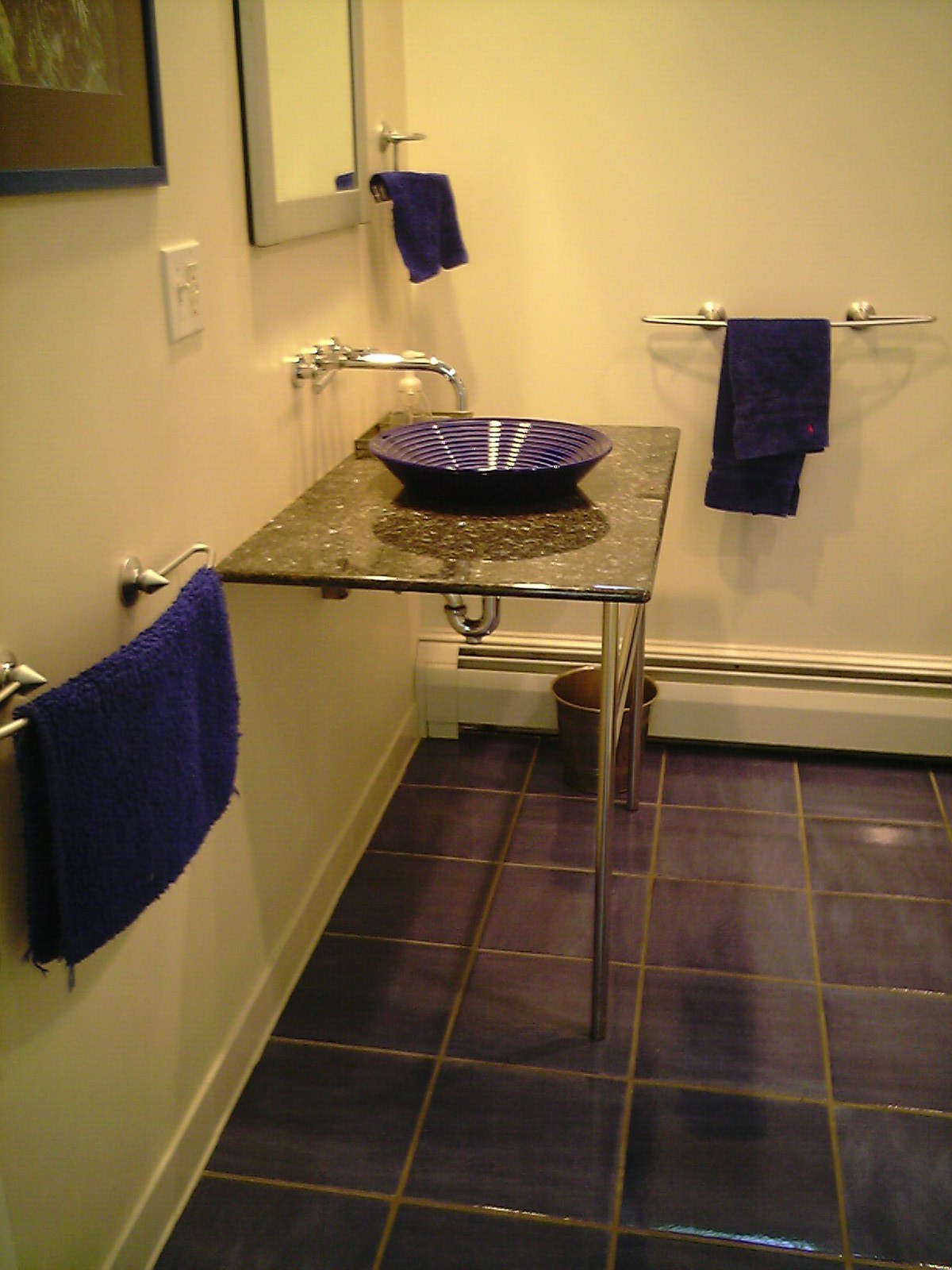The photo showcases a neatly arranged bathroom featuring a predominantly blue and white color scheme. The floor is adorned with blue tiles, which complement the white walls. At the back of the bathroom, there's a radiator with a small, bronze circular trash can positioned just in front of it. 

This bathroom is accessorized with three towels: one is hung in the center on the right-hand side of the photo, another is situated close to the entrance on the left, and a slightly smaller towel hangs on the back left wall. Above this smaller towel is a mirror with a white frame, while closer to the camera on the left side, a picture with a blue frame adorns the wall. Between the mirror and the picture frame, a white light switch is visible. 

Below this setup, a black countertop hosts a sleek sink. The sink is equipped with a silver faucet that elegantly arches over the hand-washing bowl, directing water precisely into its center. Completing this area, a visible pipe descends below the sink, guiding the water away efficiently. The detailed interplay of blue tiles, white walls, a black countertop, and silver fixtures imparts a modern and clean aesthetic to the bathroom.